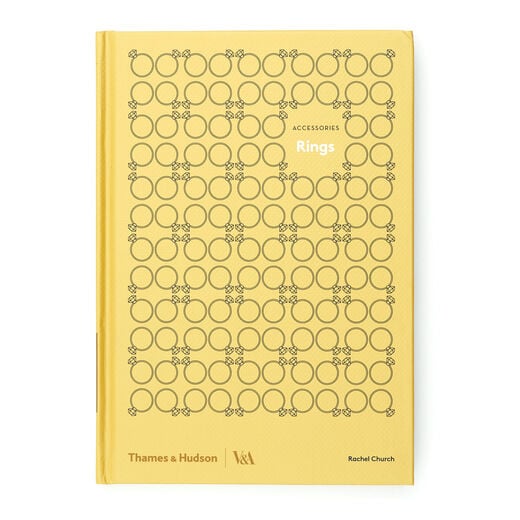The image showcases the front cover of a vintage-looking yellow hardcover book titled "Accessories: Rings." The book cover is adorned with a repeating pattern of black rings, each topped with a diamond shape, arranged in every direction—up, down, sideways—creating an intricate design. The title "Accessories" is printed in small, dark gray text, while "Rings" is displayed in slightly larger white text beneath it. At the bottom of the cover, the publisher's name, "Thames & Hudson," is written in an orange font on the bottom left, and the acronym "V&A" appears alongside it. On the bottom right corner, the author's name, "Rachel Church," is written in black. The cover design and text layout contribute to an overall appearance reminiscent of library books from the 1980s.